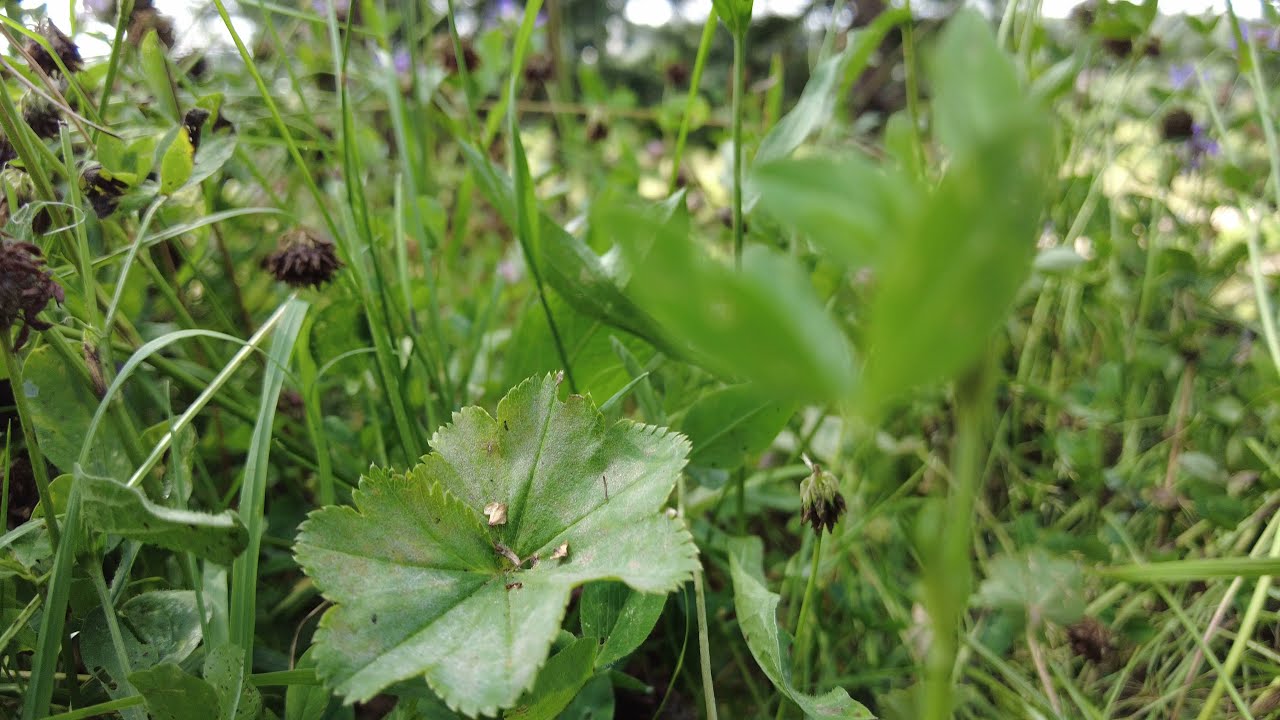This photograph, taken in a landscape orientation, is an extreme close-up of lush green plants set against a slightly visible, bright, and potentially cloudy sky. Dominating the lower left-hand corner, the photo focuses on a medium green, flower-shaped plant accompanied by a frond of fern. Surrounding this central detail, the scene is a tangle of wild greenery, including blades of grass and small purple wildflowers, some budding and others starting to bloom. There are also four or five dead flowers on the very left side. The background remains out of focus, hinting at potential buildings and blossoms in light yellow, contributing to a sense of depth. The overall scene conveys a natural, possibly wild garden setting, captured in a realistic photographic style, filled with rich greens and natural textures.